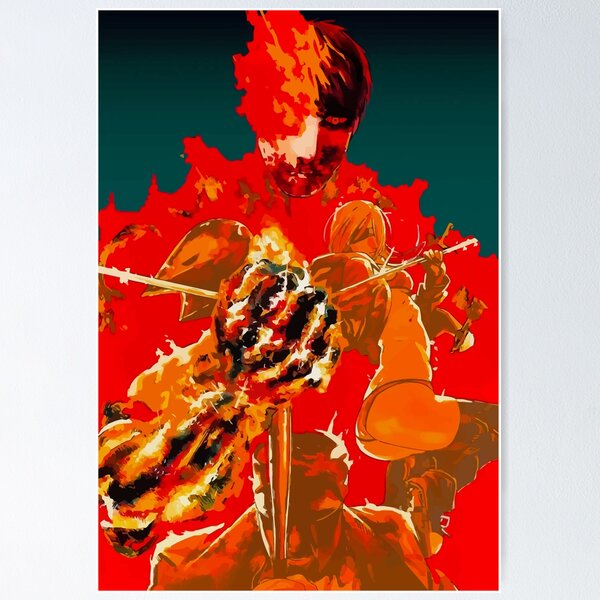The image is a dynamic, fiery digital art print displayed against a gray wall, interspersed with hues of blue and teal. It portrays an abstract yet vivid scene dominated by red flames and intricate characters.

In the foreground, a central figure draws attention: a man with a striking dual-toned hairstyle, split between normal brown on the right and fiery orange-red on the left, where it morphs into blazing flames. His face is angled downward, shadowed to hint at a beard or mustache, and his red eyes stare intensely at the viewer. His right fist is engulfed in yellow and orange flames, clenched around what appears to be three sword-like blades and a brown cylindrical object that extends downward, resembling an old-fashioned cane.

Adjacent to this flaming figure is a blindfolded woman who exudes a warrior-like presence. She is clad in a bikini, thigh-high boots tied with laces, and a short jacket. Her posture suggests she is prepared for combat, wielding a thin blade or spear-like weapon that also emanates flames. Her character is prominently highlighted by grayish hair.

In the lower portion of the image, the scene becomes a chaotic blend of black, red, and orange hues, echoing the tumultuous energy of the flames above. A repetition of the main man's image appears here, holding the brown cylindrical object now devoid of flames, positioning it across his face. Additionally, another figure emerges at the bottom, similarly posed with a clenched fist and clad in a jacket reminiscent of the main fiery figure.

Overall, the composition melds elements of anime and digital art to create a vivid portrayal of characters engulfed in an abstract, fiery aura, evoking a sense of intense action and supernatural power.